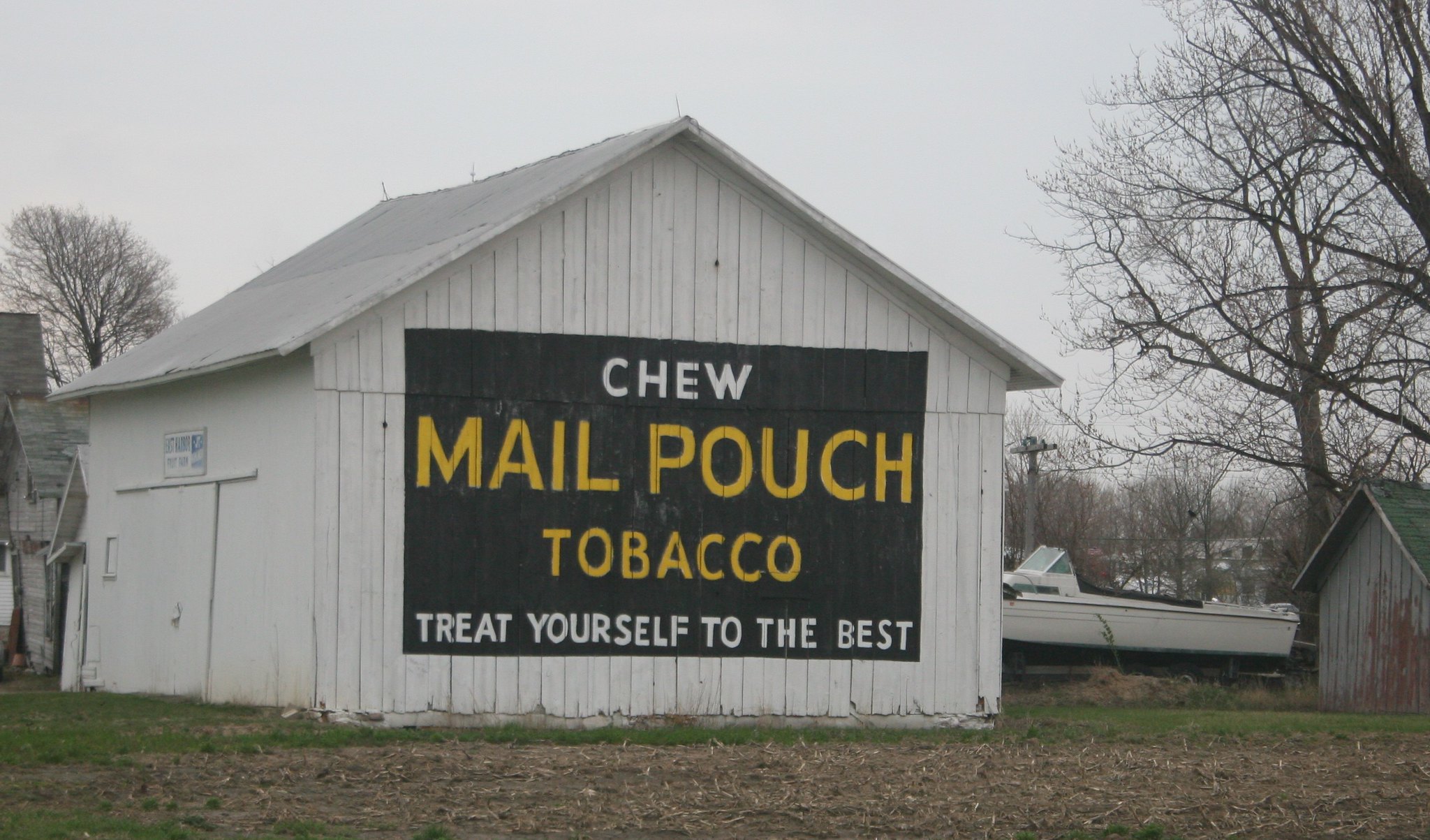The image depicts an overcast outdoor scene featuring a predominantly white barn with a matching white roof and sides. A striking black rectangular section on the end of the barn bears an advertisement painted in large, yellow and white text. The message reads, "Chew Mail Pouch Tobacco," with the tagline "Treat yourself to the best" at the bottom in white letters. The barn lacks windows and its walls are made of planks of wood nailed together. To the right of the barn, a white motorboat, possibly a ski boat with a small windshield for the pilot, rests on the ground. The surrounding area features a mix of dirt, dried grass, and patches of green grass, while leafless deciduous trees stand in the background. Additionally, off to the far right, there is a smaller shed with a green roof and gray walls.